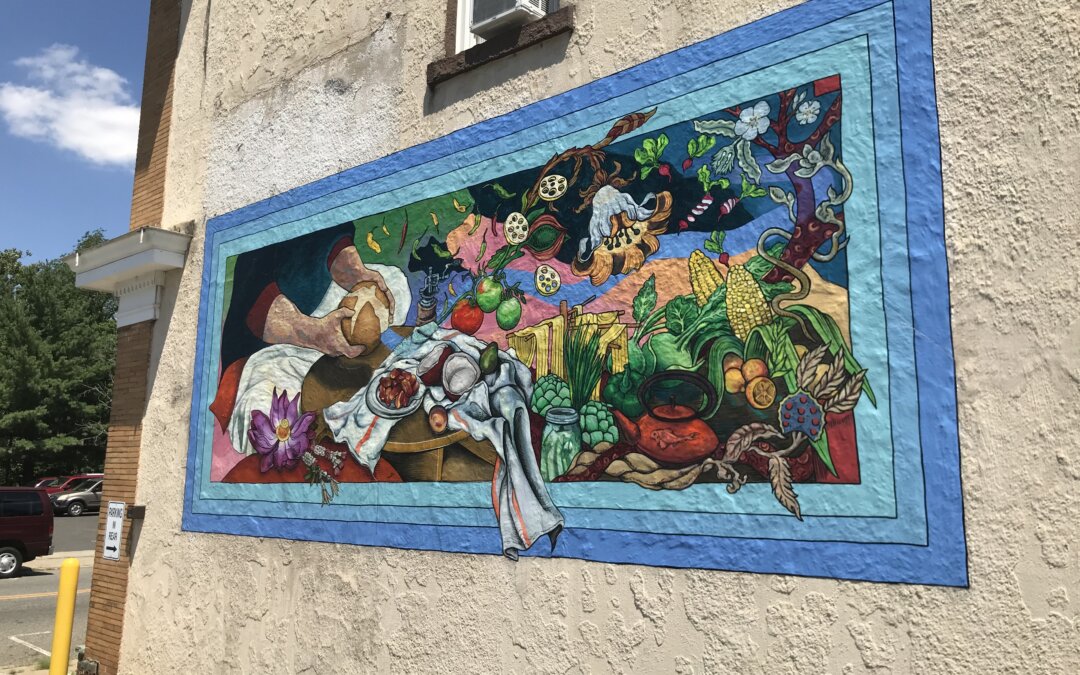This photograph captures a vibrant outdoor scene centered on a mural painted on the side of a light beige stucco building. The rectangular mural is framed by three progressively lighter blue lines. Dominating the mural is an array of colorful, detailed imagery: a brown table adorned with multicolored tablecloths and a rich assortment of vegetables, fruits, and flowers. Visible items include corn, tomatoes, oranges, pears, apples, cheese, and a teapot. On the left side, a person’s hands, clad in a dark blue garment with red sleeves, are about to break open a loaf of bread with a lighter crisscross pattern. Beyond the mural, the building features a window and light brown brickwork. The background reveals a parking lot with several cars, green trees, and a blue sky dotted with white clouds. The mural appears to celebrate the preparation of a communal meal, possibly hinting at a restaurant inside the building.